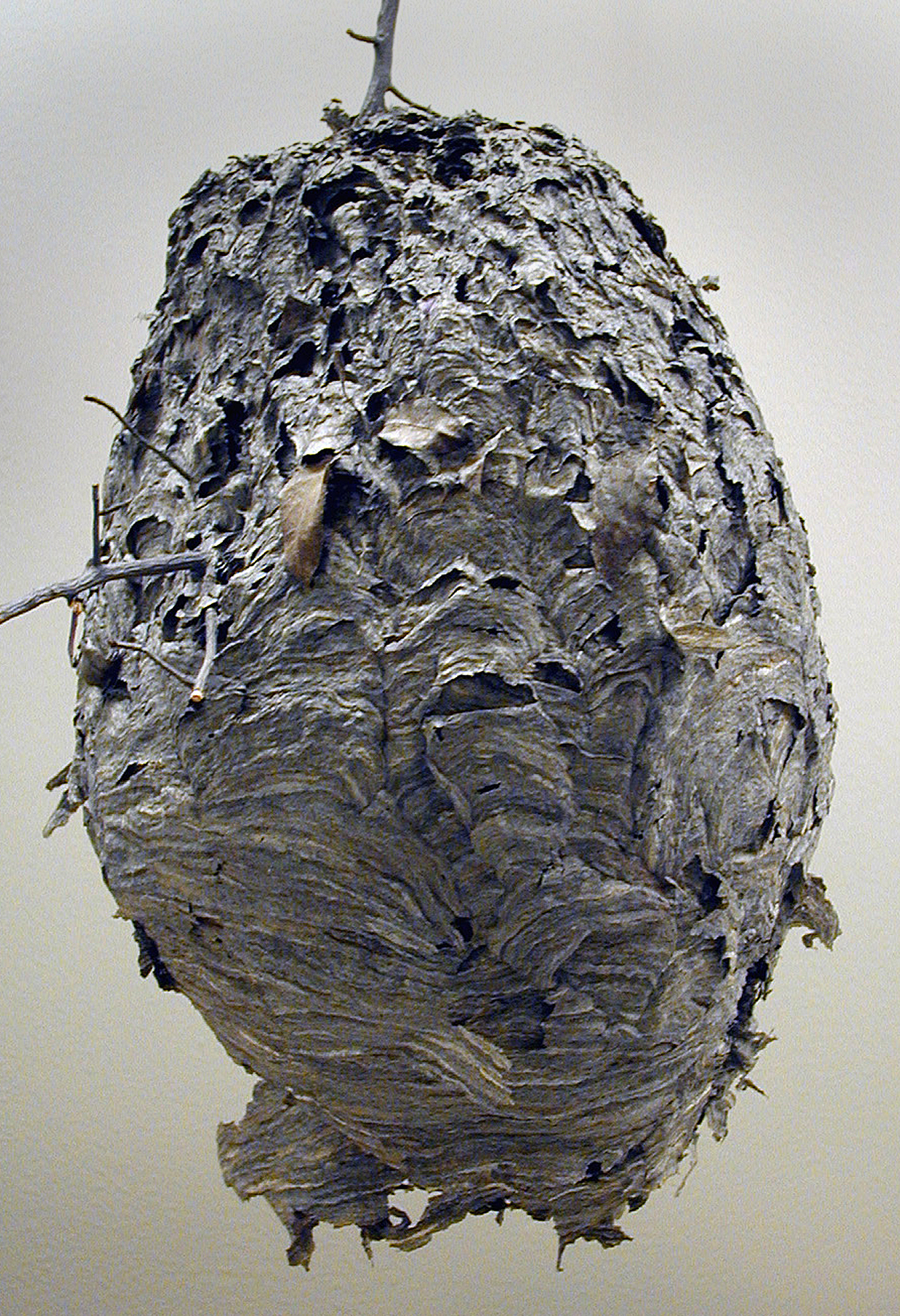This is a detailed photograph of an oblong paper wasp nest set against a plain, blurry grey and white background, likely a wall. The nest itself has a distinctive striped and mottled grey and brown texture, with parts of it peeling off on the right and left sides. The bottom of the nest shows more pronounced striping, while the top appears messier and features numerous small holes. Notably, there's an S-shaped hole in the top left and several pockmarked holes on the top right. A brown leaf is attached near the left of the center, close to one of these holes. Sticks protrude from various parts of the nest, including one emerging from a hole on the left side and another sticking out from the top. The overall appearance suggests a layered, paper-like construction typical of wasp nests.